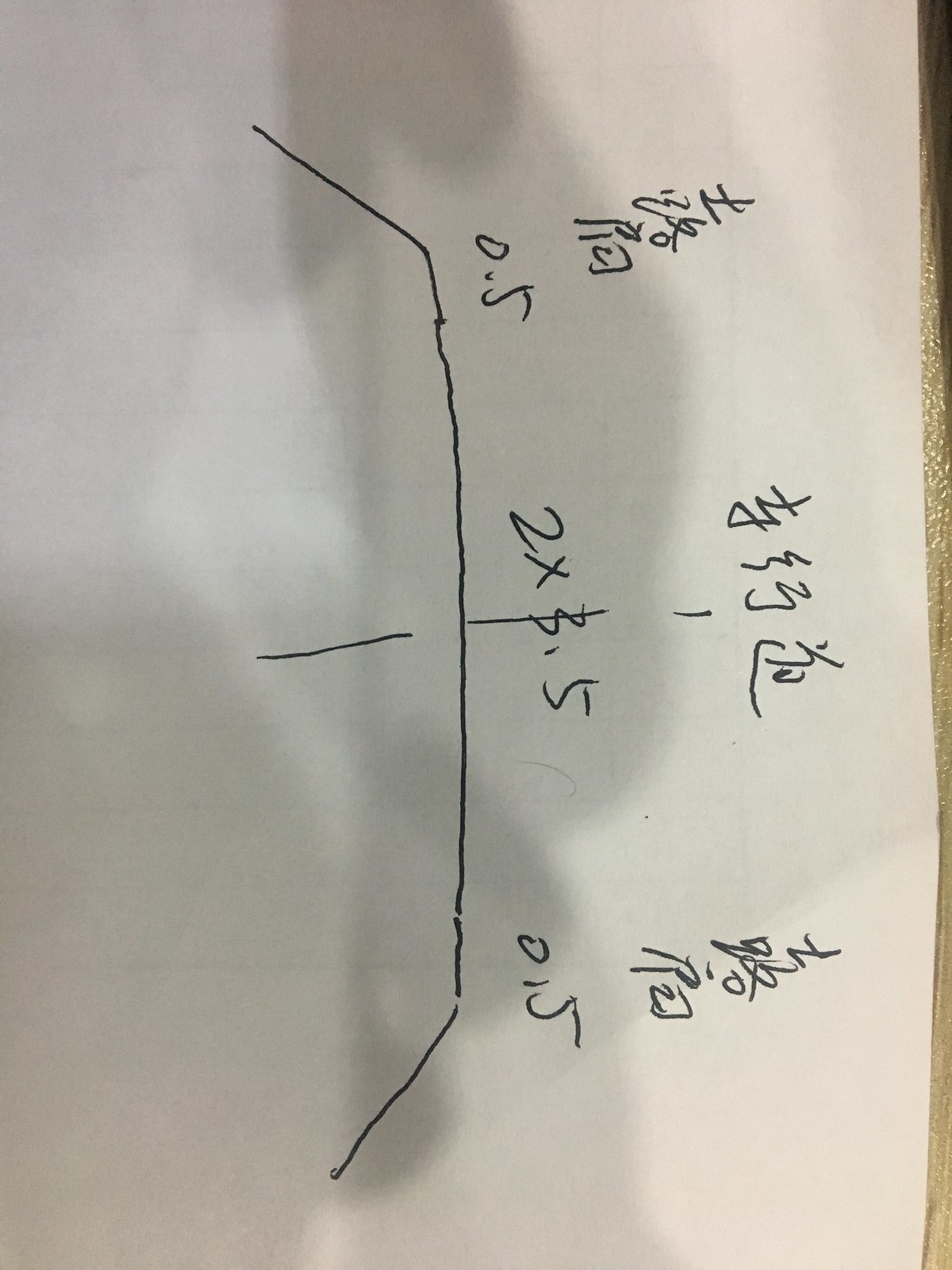This vertical photograph captures a horizontal sheet of white paper inscribed with a diagram and text in what appears to be Japanese or another East Asian script. The text is arranged in three columns at both the top and bottom of the diagram. At the center-right of the page, four characters are prominently displayed across a middle section. The hand-drawn diagram resembles a backward 'C' with its upper and lower arms bent upwards and downwards, respectively, facing the left side of the image. A line runs vertically through the center of the diagram, followed by a dash, and then another vertical line extending below. No text appears beneath this figure. Markings on the page include "0.5" at the very top-right corner, "2x3.5" in the center, and another "0.5" at the bottom-right corner of the paper. Overall, the intricate details and foreign script suggest that the document might be a technical or instructional chart, though its exact purpose remains unclear due to the language barrier.